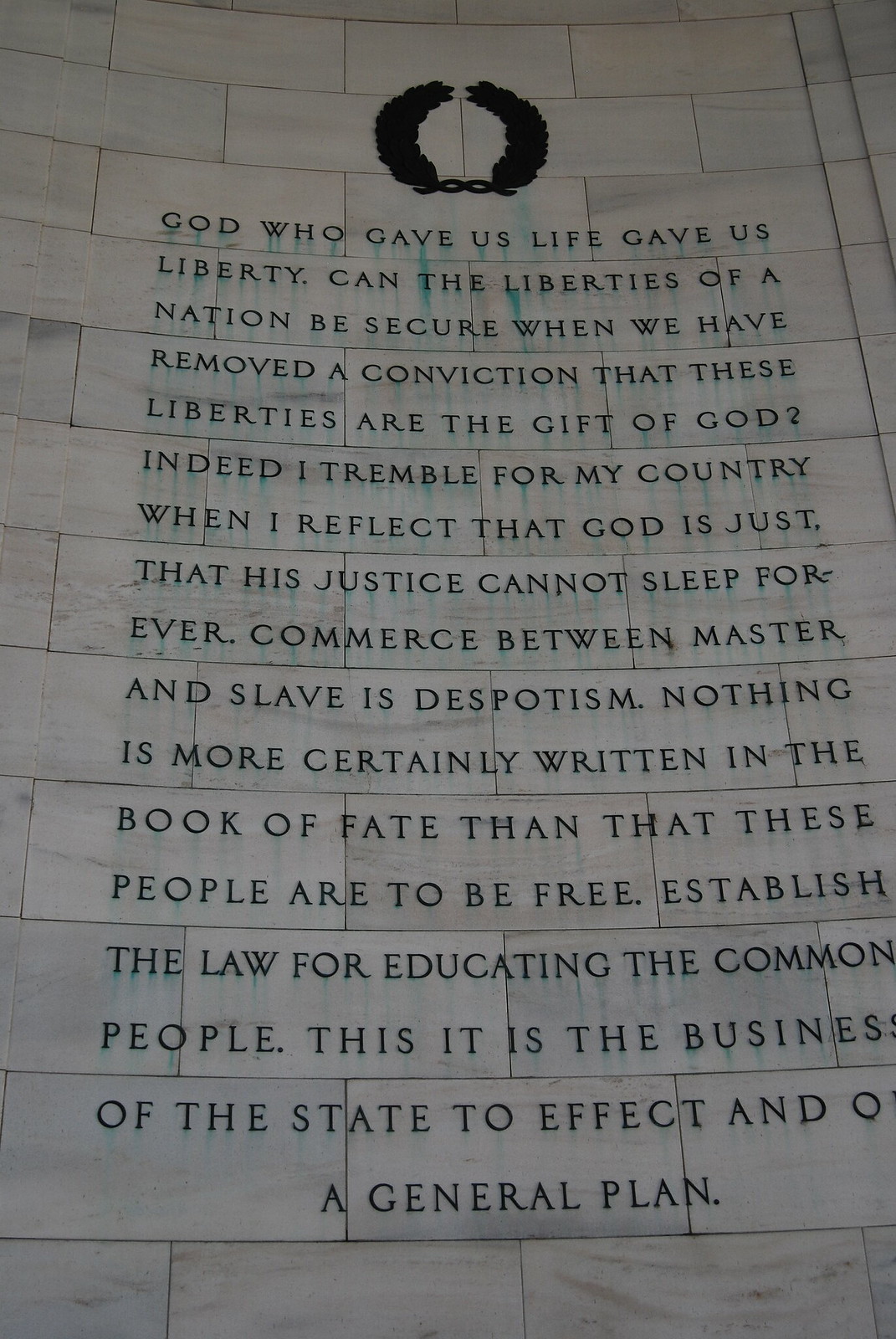This image depicts an inscription on what appears to be a memorial wall made from white marble or stone bricks. The tall, vaulted wall prominently features a black illustration of wings or a wreath at the top. Below this, an extensive inscription is etched in black capital letters, which reads: "God who gave us life gave us liberty. Can the liberties of a nation be secure when we have removed the conviction that these liberties are the gift of God's? Indeed, I tremble for my country when I reflect that God is just, that his justice cannot sleep forever. Commerce between master and slave is despotism. Nothing is more certainly written in the book of fate than that these people are to be free. Establish the law for educating the common people. This is it, the business of the state to effect and the general plan." The setting appears to be the interior of a historical site or a memorial, possibly similar to the Lincoln Memorial.